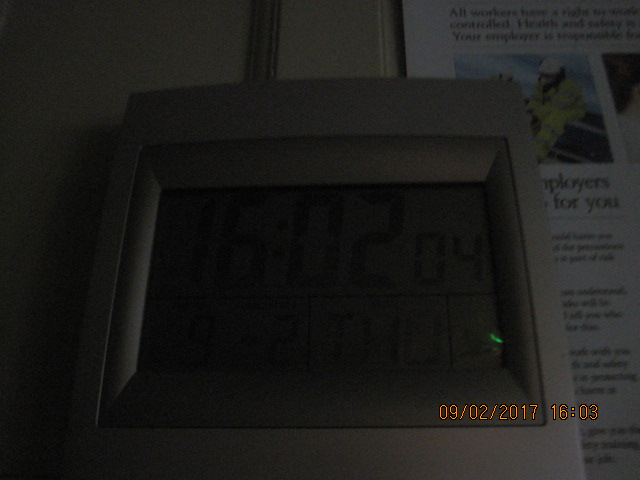In this dark and dimly lit photograph, we observe a low-resolution image depicting a gray thermostat affixed to a gray wall. The bottom right corner of the image features the timestamp "09/02/2017" in orange print, with the time marked as 16:03. To the right side of the wall, there appears to be a poster, possibly a safety notice, though the full details are not entirely legible. The poster contains black print with the partially readable phrase "employers for you." It also includes an image of a person dressed in a yellow outfit, reminiscent of attire worn by rescue workers or firefighters.